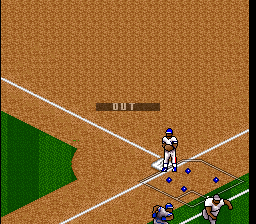In the bottom right corner of the image, a group of baseball players can be seen. One player is standing on a base while another, presumably the pitcher, is positioned nearby. The players are dressed in white uniforms; one is wearing a blue hat and another a white hat. The field itself is predominantly brown, with scattered patches of green grass visible in the bottom right and bottom left corners. Dominating the center of the image is the word "OUT," indicating that the image was captured during a play resulting in an out or a ball going out of bounds. The upper portion of the image is entirely brown with no additional elements or details.